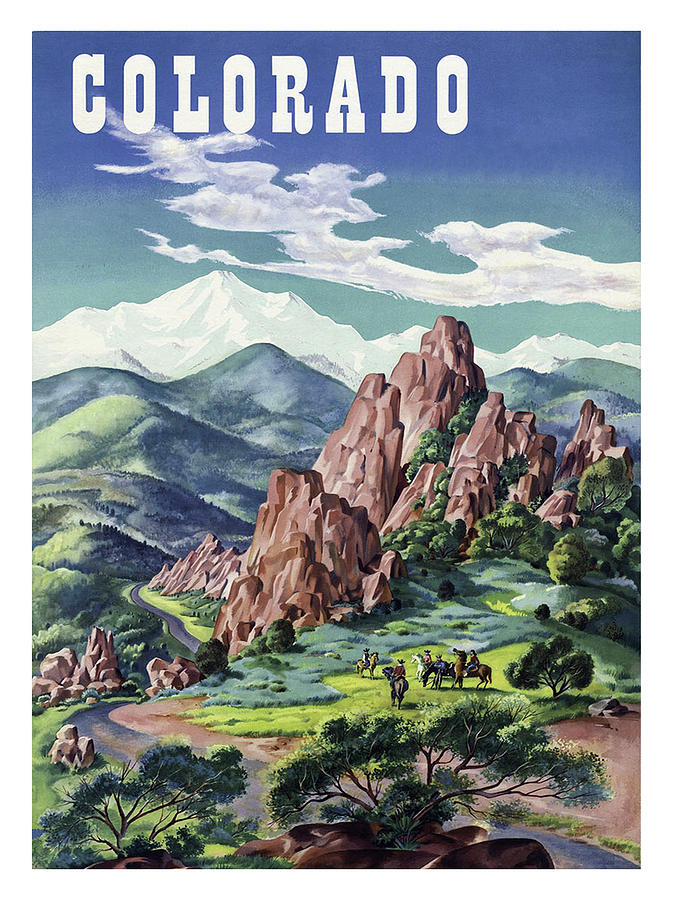This vintage-style poster features a striking, historical illustration of Colorado. Dominating the top of the poster, bold white uppercase text reads "Colorado" across a vibrant sky that transitions from a deep royal blue at the top to a turquoise blue lower down. Wisps of white clouds float in the sky, adding to the scenic beauty. 

Below, the landscape showcases a majestic mountain range capped with white snow, likely representing the Rocky Mountains. Descending from these lofty peaks, the terrain gradually shifts from additional blue-toned mountains to lush, green lower elevations. The green hills expand towards the foreground, dotted with trees and patches of brown dirt and soil.

In the lower part of the image, a winding road snakes around a rocky outcrop reminiscent of the Garden of the Gods Park, complete with sparse green bush vegetation. At the base of this rocky formation, five or more horseback riders navigate the beaten path, set against a serene backdrop of expansive hills and intricate landscape details.